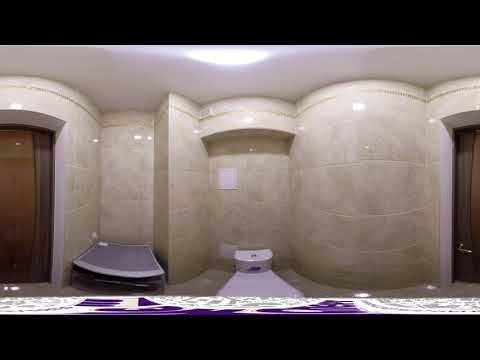The image is a 360-degree interior view of a bathroom. The fisheye or wide-angle lens creates a skewed effect, distorting the perception of the room. The walls are covered in light, shiny stone tiles with a yellowish-white hue, giving them a marble-like appearance. The white ceiling features a light that reflects off the glossy tiled surfaces. There are two wooden doors, one on the left and another on the right, both displaying dark brown textures.

Prominently in the center of the image is a white toilet with a semi-circular top. Below the toilet is a long white rectangle with purple letters, which appears distorted due to the lens. A piece of paper or poster is visible on the wall behind the toilet. On the bottom left of the image, there's a square table or platform situated in a corner of the bathroom. Despite some ambiguity due to poor image quality, the overall scene is a detailed depiction of a modern, glossy-tiled bathroom with reflective surfaces and multiple wooden doors. The black border at the top and bottom of the image frames the scene, adding to the visual distortion.